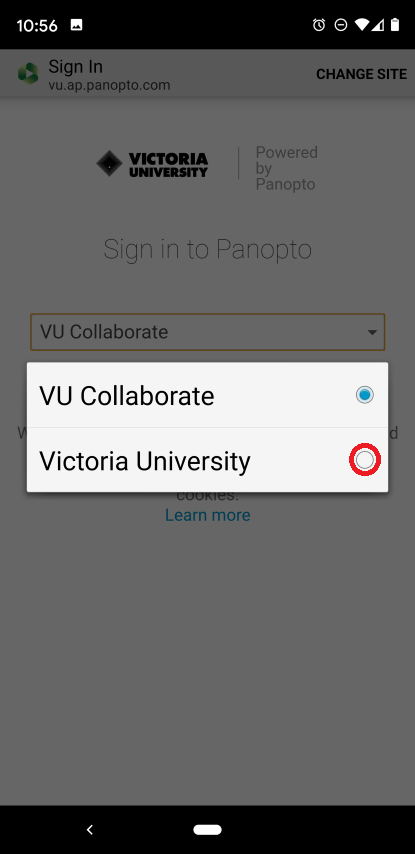A mobile screenshot depicts a user attempting to sign into an application or webpage. At the top of the screen, the phone's UI displays the time as 10:56 on the left side, accompanied by a screenshot notification. On the right, a series of icons are visible: a timer, a circle enclosing a minus sign, Wi-Fi, mobile data, and a battery icon that appears to be between 80% and 90% charged.

The main content of the screenshot shows an app interface with the heading "Sign In" and the URL vu.ap.panopto.com at the top. To the right, in bold letters, the option "Change Site" is available. Below this, it reads "Victoria University, powered by Panopto." The next line prompts the user with "Sign in to Panopto," followed by a dropdown menu.

A pop-up menu obscures the rest of the page content, offering two sign-in options: "VU Collaborate" and "Victoria University." The option "Victoria University" is highlighted with a red circle to indicate user selection, while the currently selected option, "VU Collaborate," is shown active in the screenshot. At the bottom, partially obscured by the pop-up, there is a hyperlink labeled "Learn more."